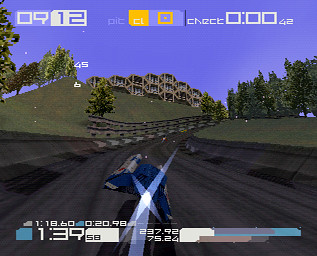The image is a screenshot from a video game that features a futuristic blue and white flying car emitting a jet trail from its back. The car hovers slightly above a recessed gray track that stretches forward and curves to the right. Arrows line the left side of the track, which is flanked by trees with green leaves. Above the track stands a tall, pyramid-shaped structure. The scene includes additional elements: across the top of the screen, there are numbers in white on a blue sky background, and in the center, there's a notable yellow figure, potentially a square with a yellow dot inside. The bottom part of the screen displays several game statistics, though their specifics are not labeled. The countryside setting also hints at poorly rendered mountains and additional greenery, adding to the immersive gaming environment.